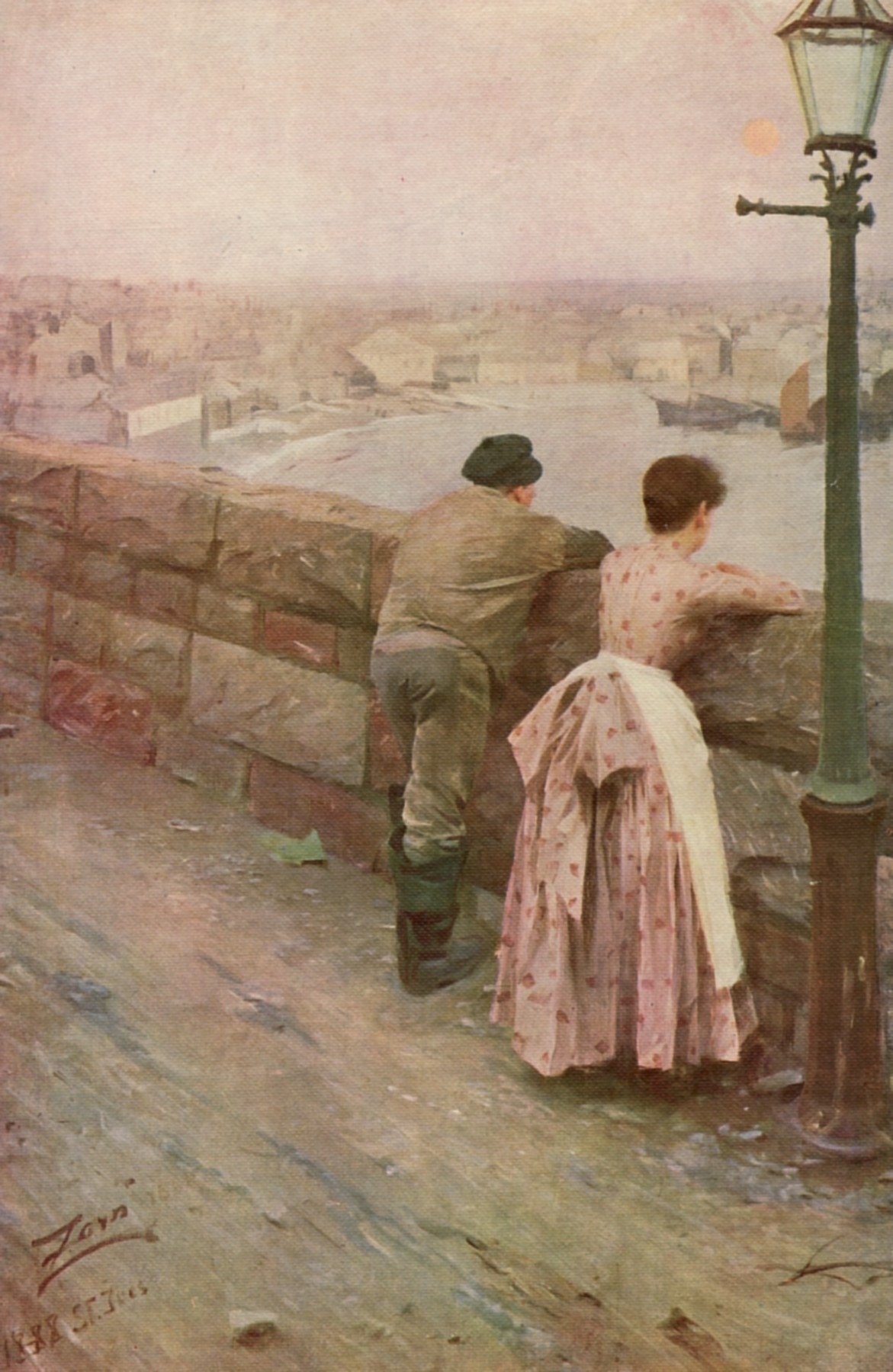In this oil painting by Anders Zorn titled "Fisherman at St. Ives" from 1888, the scene captures a realistic and muted depiction of a man and woman with their backs turned, leaning on a heavy stone wall that overlooks a river and a fading village in the background. The woman, standing next to a tall outdoor lantern on the right, is dressed in a light pink, long-sleeved dress adorned with red designs, and her hair is neatly tied up. She also wears a white apron, and her arms are crossed as she leans on the wall. The man, positioned to her left, dons a brown jacket, light-colored pants, knee-high black boots, and a black hat. Both appear to be gazing out at a circular bay dotted with fishing boats, symbolizing a connection to the man's occupation as a fisherman. The muted colors of the painting – dominated by grays, browns, light greens, and pinks – evoke a somber and reflective mood. At the bottom left corner, a signature or name, possibly "F-O-R-N," along with the numbers "1888," is faintly visible, adding an additional layer of historical context.